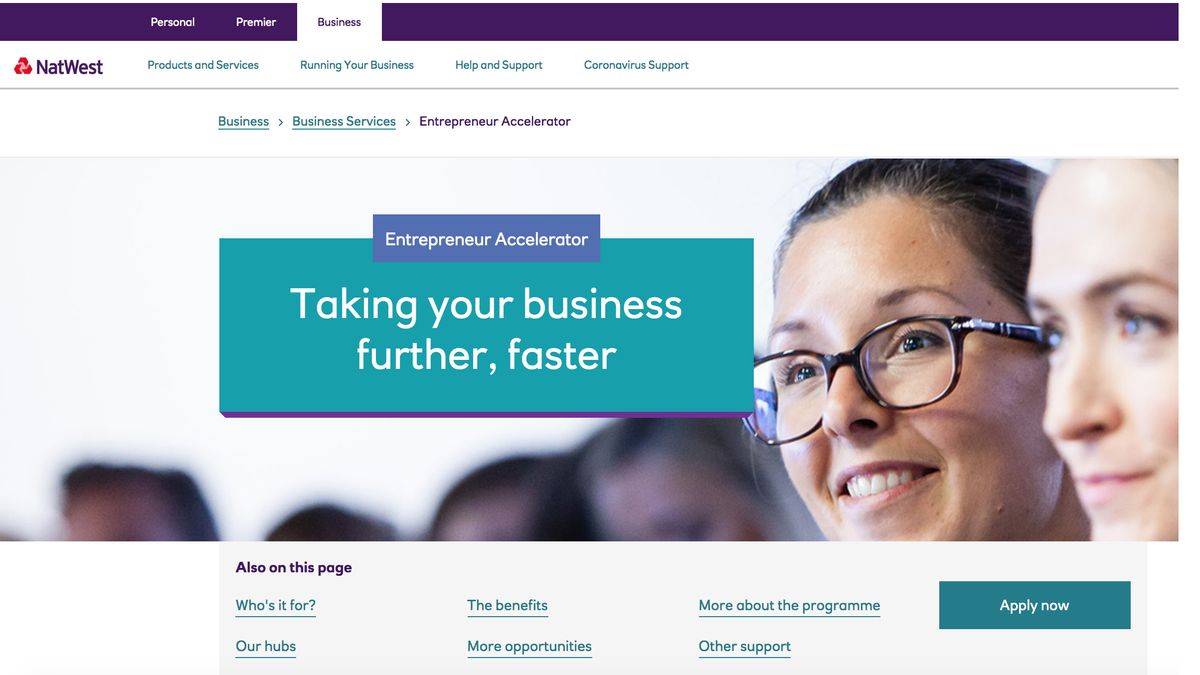This detailed caption provides a comprehensive description of the visual elements and layout found within the image:

At the top of the image, there is a purple horizontal rectangle featuring white text that reads "Personal," "Premier," and "Business." The "Business" option stands out with white text on a purple background, indicating it is the selected category. Below this, a red logo is positioned next to the text "NatWest" in purple. Following this, in blue-green text, various sections titled "Products and Services," "Running Your Business," "Open Support," and "Coronavirus Support" are listed.

Continuing down, in the same blue-green text, it reads "Business" with a right-pointing arrow, followed by "Business Services" with another right-pointing arrow. The text "Entrepreneur Accelerator" appears in purple lettering.

The image below these text elements features a layered design with a prominent blue rectangle containing the words "Entrepreneur Accelerator." Beneath this is a larger green-blue rectangle displaying the message "Taking Your Business Further Faster." These text blocks overlay the underlying photograph.

In the photograph, two women are situated near the right side; one wears glasses while the other does not. The background is slightly blurred, revealing indistinct shapes that suggest the presence of additional people.

At the bottom of the image, a series of text options are listed with the same blue-green coloring: "Who's It For," "Our Hubs," "The Benefits," "More Opportunities," "More About the Program," "Other Support," and an "Apply Now" button.